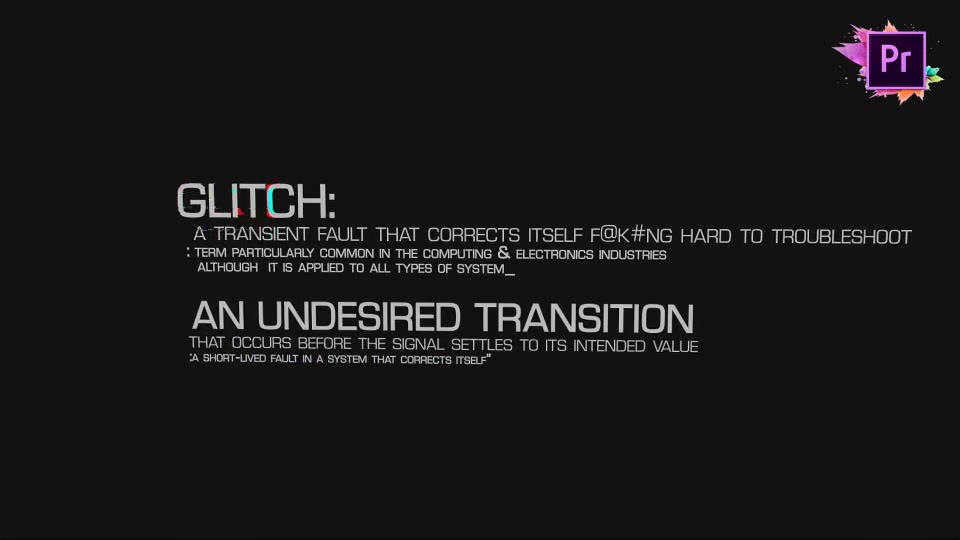The image is predominantly a black rectangular background with a cluster of detailed text centrally positioned. In the upper right corner, there's a small logo featuring a blue-outlined square enclosing the letters "Pr" in blue, set against a black background with hints of yellow and blue leaf patterns behind it.

Directly in the center of this image, bold gray text declares "Glitch:", followed by the description in a skinnier gray font: "a transient fault that corrects itself, fucking hard to troubleshoot, a term particularly common in the computing and electronics industries, although it is applied to all types of systems." Beneath this, another bold gray heading states "An undesired transition," with additional skinnier text explaining "that occurs before the signal settles to its intended value. A short-lived fault in a system that corrects itself." 

The design elements and the technical language suggest an educational or presentation setting, and the image employs a palette of black, gray, blue, yellow, and hints of purple, pink, orange, and green.